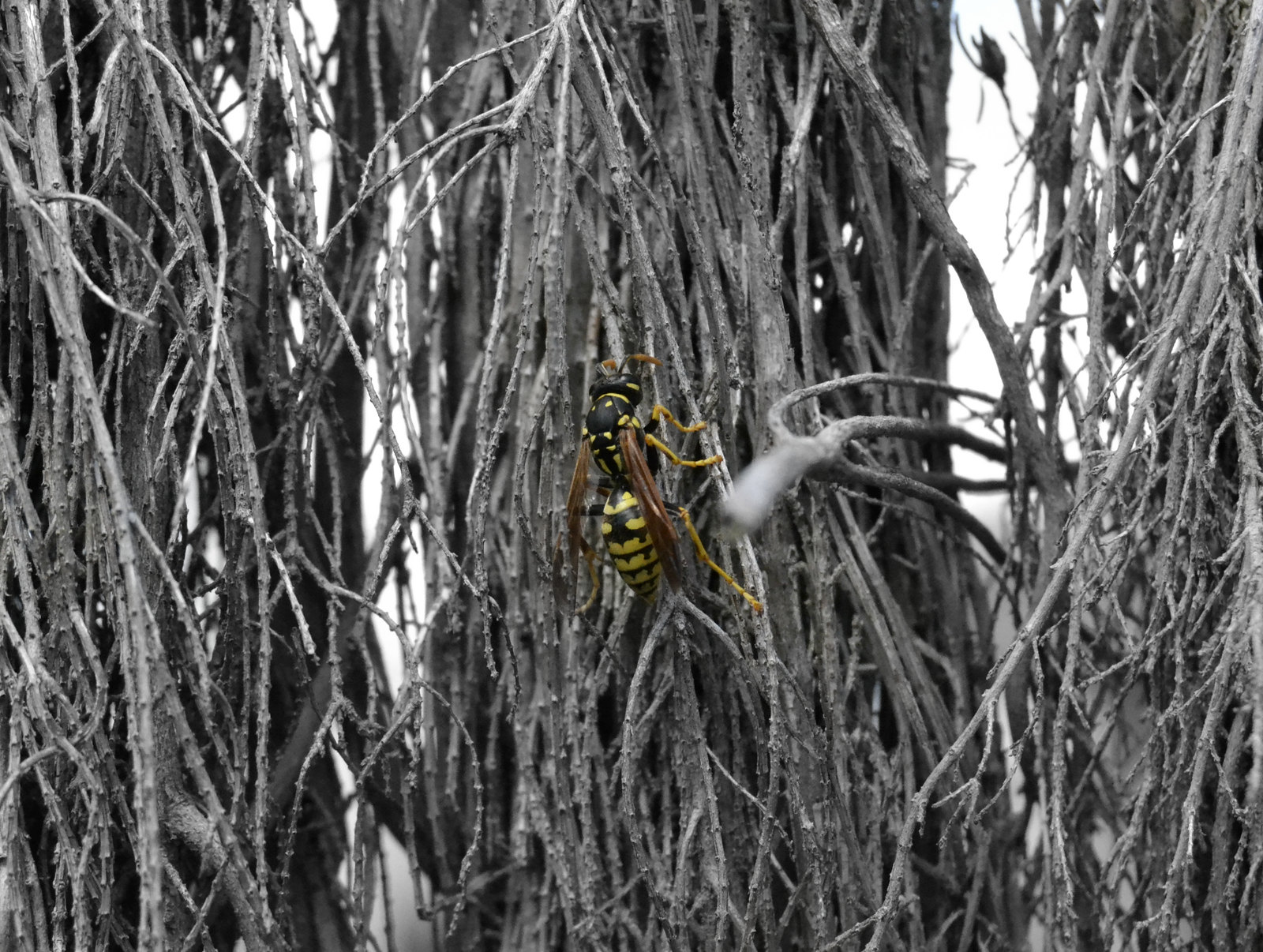In this strikingly edited black and white photograph, the central focus is a vividly colored wasp. The wasp, with its distinct black and yellow stripes and brown wings tightly folded, stands out starkly against a dense backdrop of old, seemingly lifeless vines and branches. This monochrome background, suggestive of dying trees with thin, stick-like branches, emphasizes the wasp’s fresh, vibrant appearance. The sky peeking through the dense plant life is a solid shade of grayish white, enhancing the muted, somber mood of the scene. The wasp, positioned in the center and appearing to cling to a vine, seems to be either searching for something or resting. Its stinger is faintly visible, and its long yellow legs add to its striking presence. The detailed focus on the wasp amidst the creatively desaturated landscape highlights the contrast between life and decay in this visually captivating image.